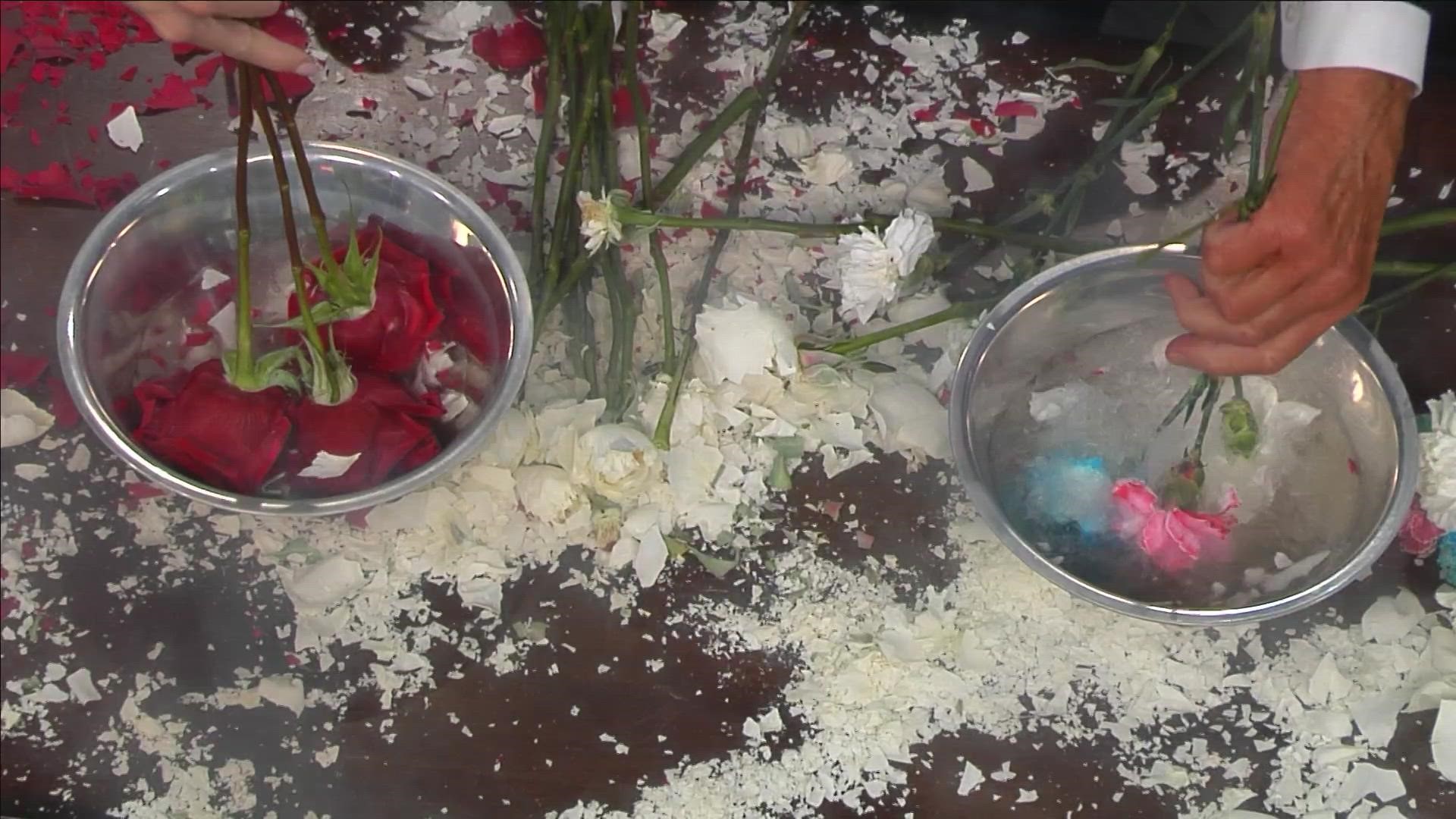The image captures a detailed scene on a brown wooden surface, likely a tabletop. Scattered across the table are broken petals and stems, predominantly from red roses, creating a delicate yet chaotic arrangement. Centered on the table are two silver bowls filled with icy water, each attended by a pair of hands. On the left, a woman's hand holds three vibrant red roses, submerging them into the water. On the right, a man's hand, distinguished by a white cuff, dips a trio of flowers—one blue, one pink, and one white—into the other bowl. Between the bowls lies a cluster of intact white flowers, adding a contrast to the fragmented beauty surrounding them. The scene suggests an artistic or preservation process, with bits resembling paper or eggshells interspersed among the floral fragments.